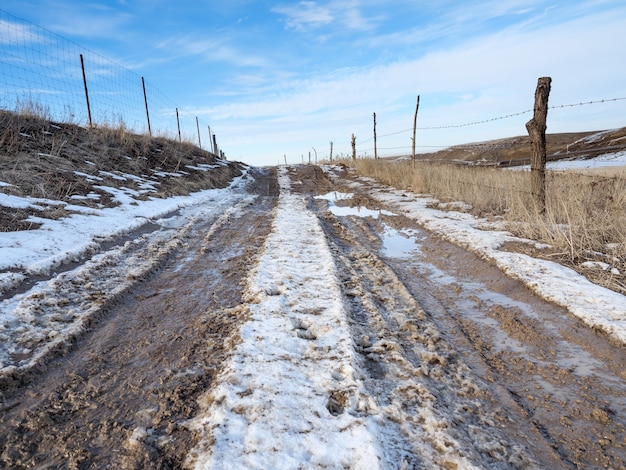The image depicts a rugged country road in what appears to be wintertime in Wyoming, beneath a clear blue sky adorned with wispy cirrus clouds. The road is a muddy dirt track, deeply rutted with tire tracks, and interspersed with patches of melting white snow. Down the center of the road, where no tires have passed, the snow appears more prominently but is mixed with mud, creating a slushy path. Barbed wire fences with wooden posts flank both sides of the road, standing amidst dry, brown grass and weeds, contributing to the desolate winter landscape. Puddles formed from the melting snow dot the road, adding to its wet, rugged appearance. The road stretches into the distant horizon, disappearing into the hilly background, capturing the vast, open expanse typical of the rural United States.